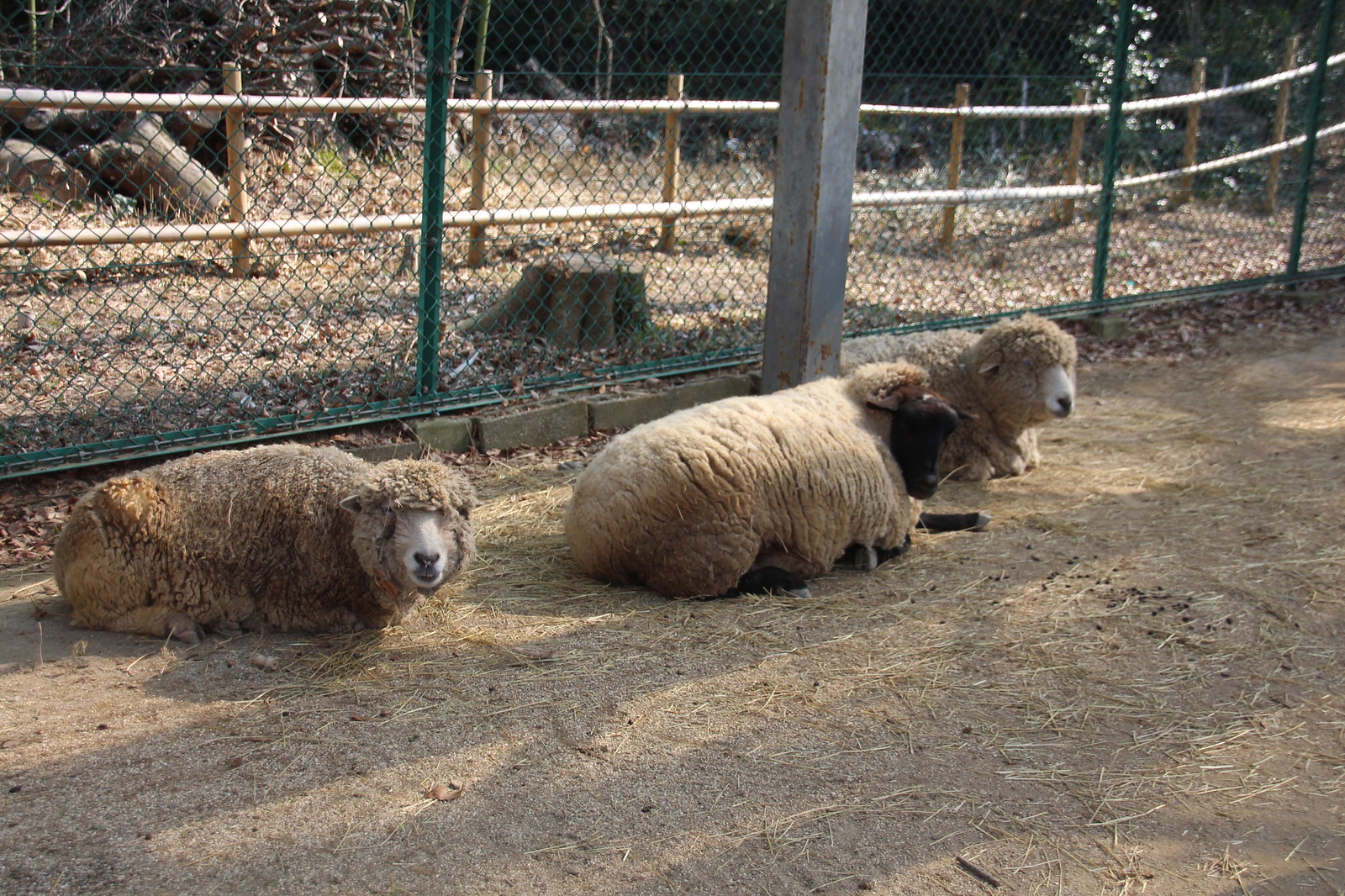In this color photograph, three sheep lie in a heavily secured enclosure that suggests a petting zoo or park setting rather than a farm. The enclosure features a chain-link fence with a rubberized green coating, reinforced by a row of unmortared cinder blocks at its base, presumably to prevent digging. Beyond this chain-link barrier, there is another row of round wooden posts connected by a top and bottom rail, acting more as a decorative boundary than a functional one. Behind these posts lies a dark wooded area scattered with brown autumn leaves.

The foreground of the enclosure is covered in bare dirt mixed with straw or hay, along with some sheep droppings, indicating a well-used area. A tree stump stands between the two fences, adding a natural touch to the otherwise structured environment. Dominating the center background of the image, a tall post, possibly wooden or concrete, rises and extends out of frame.

The three sheep, all with dirty, matted brown fleeces, are positioned with their bodies parallel to the right-hand side of the image. The sheep on the left looks directly at the camera, revealing a white face contrasted by its brown body. The center sheep, distinguishable by its black face and legs, also faces right but remains in clear view. The third sheep, mostly obscured by the others, similarly faces the right side of the image, sharing the white-faced characteristics of the first. The overall scene depicts a serene moment of repose within a well-contained and naturalistic setting.